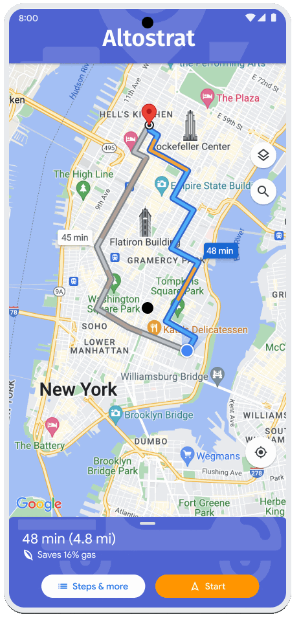A detailed map displayed on a smartphone screen provides navigation directions from a current location to Hell's Kitchen, New York. The top of the screen prominently shows the app name "Alto Strat". The map underneath fills nearly the entire screen, prominently marking New York City and illustrating significant landmarks and neighborhoods. The Hudson River is visible, with a stair-step pattern indicating the suggested route.

Hell's Kitchen is clearly marked with a red pin, standing out as the destination. Key areas like the High Line, Lower Manhattan, Soho, Washington Square Park, and the Delicatessen are identifiable on the map. Other notable locations such as Brooklyn Bridge Park, Fort Greene Park, the Plaza, and Rockefeller Center are also visible.

At the bottom of the screen, the map reveals the route details: the distance to Hell's Kitchen is 4.8 miles, estimated to take 48 minutes. A notation indicates that following this route can save 6% on gas. The interface features a "Steps and more" section, along with a prominent orange "Start" button, inviting the user to begin navigation.

This well-illustrated navigation map not only guides the user through the bustling streets of New York but also highlights the efficiency and savings of the proposed route.